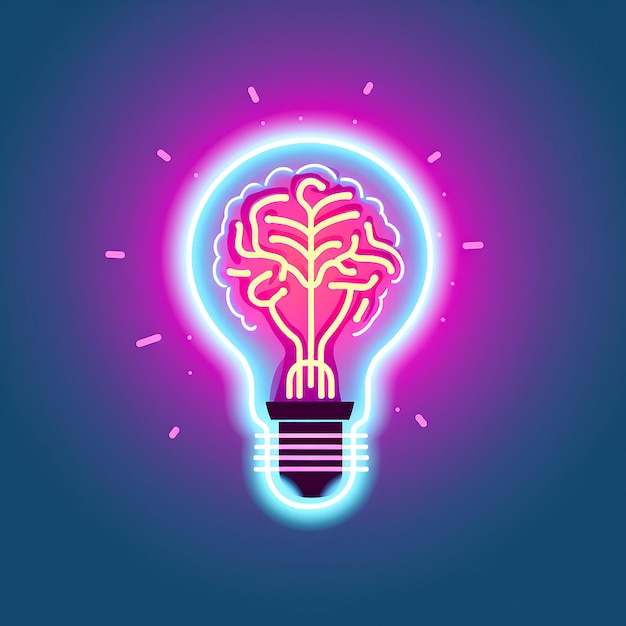This detailed image showcases a digital render of a light bulb set against a predominantly dark blue background. The light bulb radiates vibrant neon hues, with a glowing blue-white outlining its classic shape. The lower portion of the bulb is encircled by vivid purple neon light. Inside, there appears to be an intricate design resembling a human brain, composed of light-colored yellowish-orange lines that evoke the structure and texture of a brain's folds. This design is intersected by four pink horizontal lines at the bottom. The base of the bulb is black and features four horizontal bars. In keeping with a 1920s or Miami Beach 1980s neon style, the bulb is adorned with a bright purple radius and pink dashed lines surrounding it, adding to the dynamic and striking visual effect. The overall aesthetic is one of exuberant neon brilliance, combining elements of retro and futuristic design.